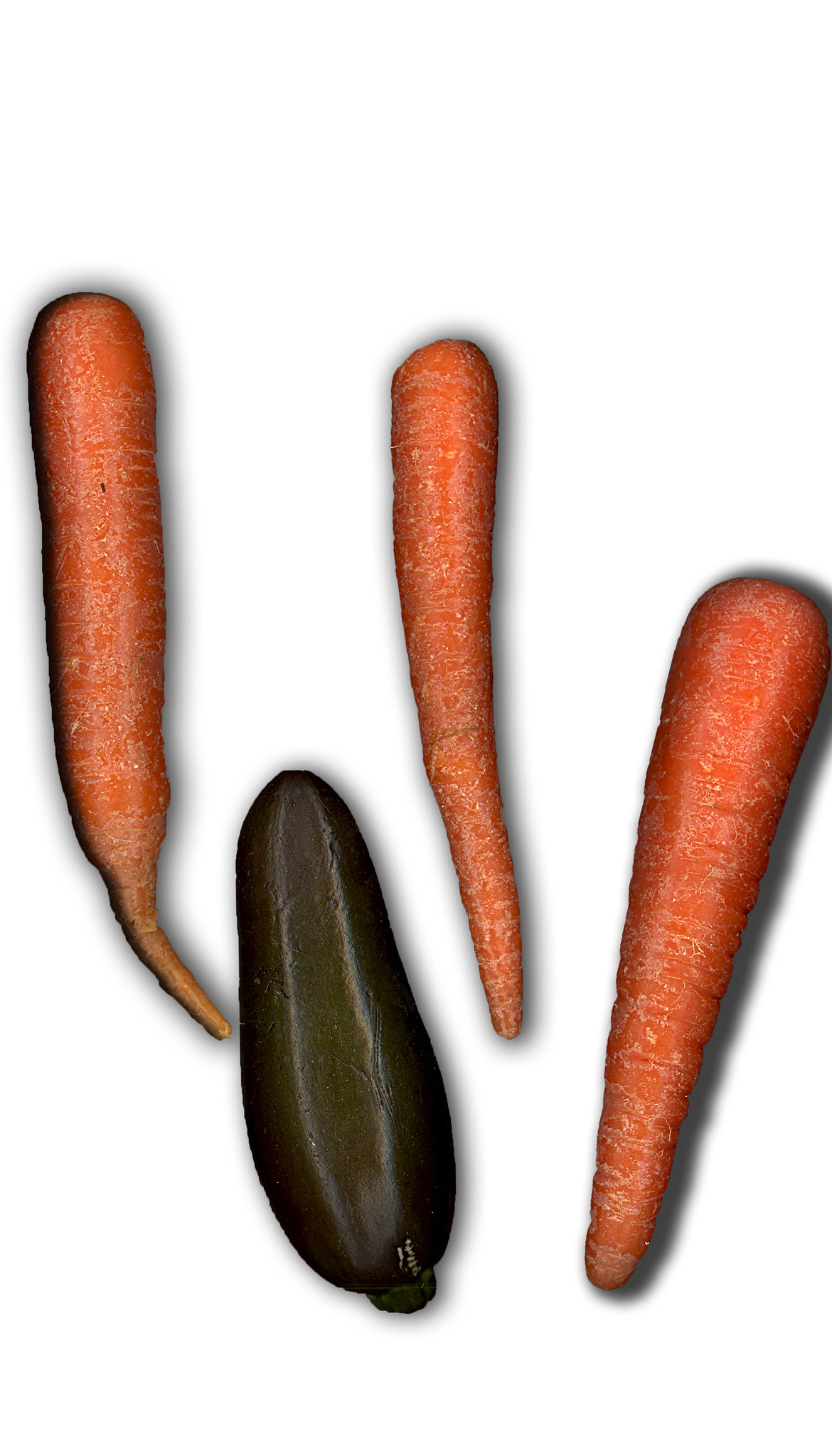The image depicts a white background featuring a close-up of three large, vibrant orange carrots and a smaller, dark green zucchini. The carrots, all pointing downward with their narrow tips, are arranged vertically from left to right. The carrot on the far left has a slight curve at its bottom end. Nestled between the second and third carrots is the zucchini, noticeably shorter and wider, with a nearly black hue and a hint of green. The vegetables appear realistic but possess a black fuzzy outline, suggesting possible computer editing or animation.